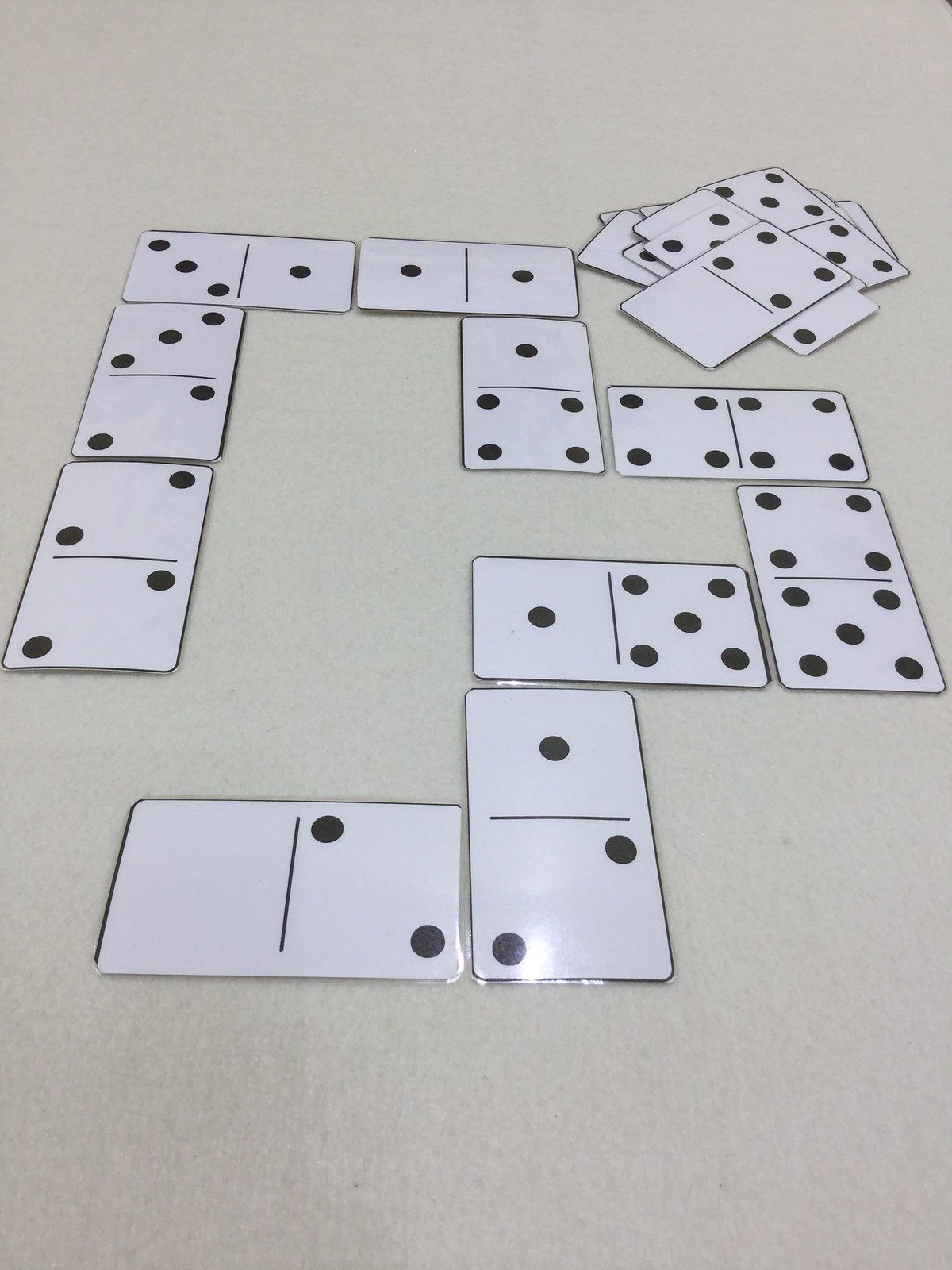The photograph, taken from a high angle, showcases a minimalist white floor devoid of any shadows. At the center of the image, there is a sequence of laminated paper dominoes, reflecting light from above. The shiny lamination gives them a slightly glossy appearance. The dominoes, arranged in a vertical line, begin with a piece showing 'blank-2', followed by '2-1', and continue in a logical sequence including '1-5' among others. In total, there are 10 to 11 dominoes laid out in this arrangement, each piece properly connected by matching sides. At the top right corner of the image, there is a small pile of 7 to 8 unused dominoes, also white with black dots. The simple, yet structured composition emphasizes the clean and orderly layout of the dominoes against the stark white background.